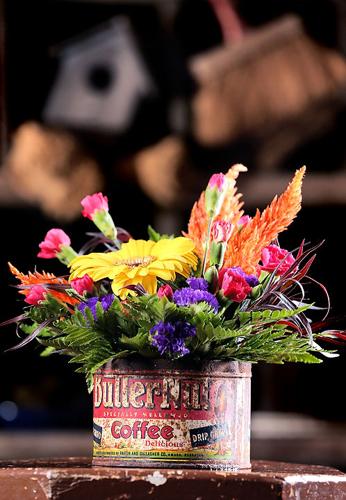A vivid and charming bouquet of flowers bursts from an old, rusted Butternut Coffee can, its vintage label featuring the words "delicious" and "drip," despite the worn and weathered state. The flowers, in hues of yellow, pink, red, orange, and purple, create a lively contrast to the verdant green leaves and stems. Nestled in the stubby, round can, the blooms cluster near its rim, complementing the can’s rustic charm. This arrangement sits atop a small, octagon-shaped wooden table, equally worn with a chipped, maroon finish. The background, though out of focus, hints at indoor elements, including a small gray birdhouse in the top left and an antique cleaning brush on the top right, adding to the scene's quaint and rustic atmosphere.